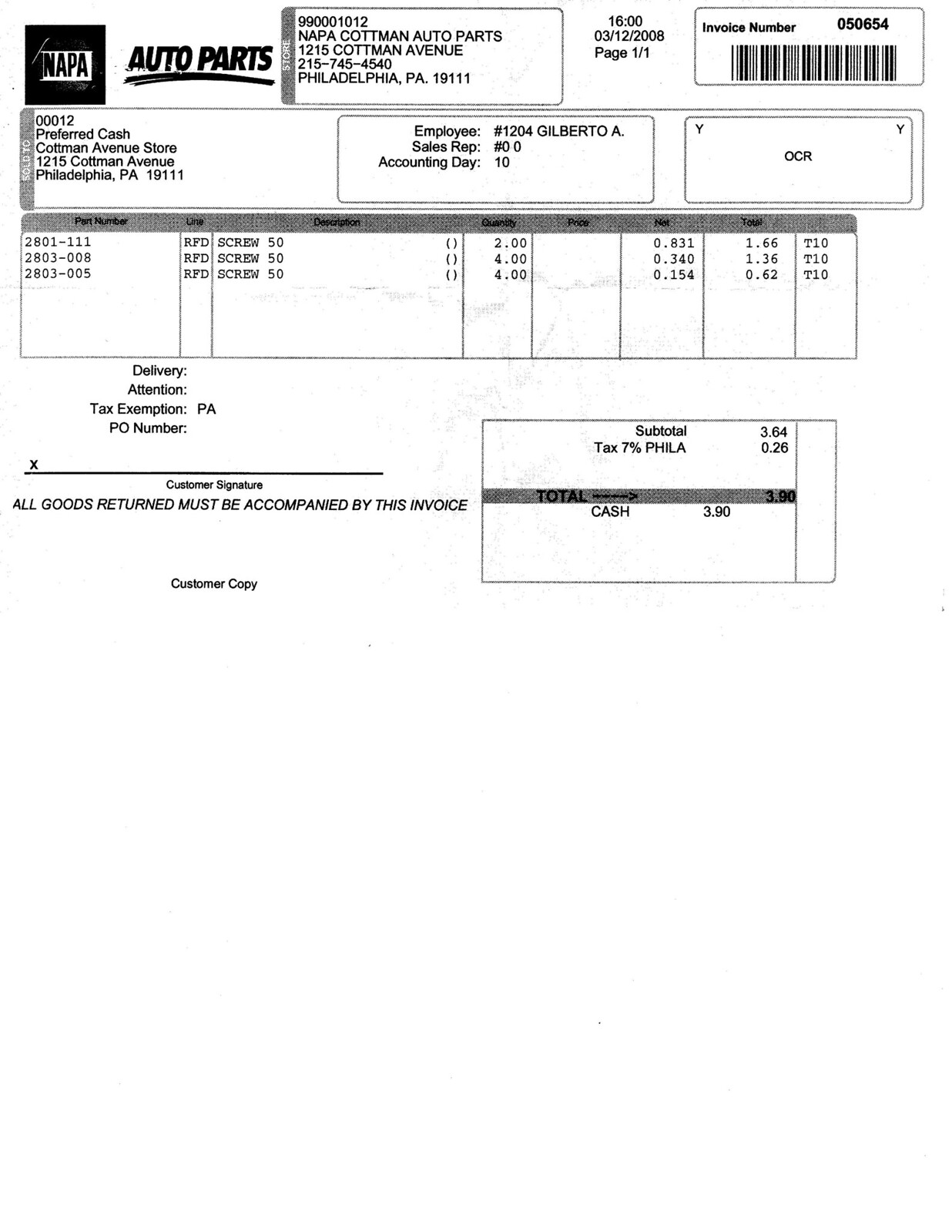This image depicts a detailed receipt from Napa Auto Parts, located at 1215 Cotman Avenue, Philadelphia, Pennsylvania. The receipt, printed on white paper with black text, is dated March 12, 2008, at 1600 hours and is labeled as page 1 of 1. The invoice number is 050654, which is displayed alongside a barcode at the top right.

The receipt is organized into several sections. At the top, it includes the store's name, address, and phone number, followed by the sold-to information. Below that, there are details about the employee who processed the transaction, identified as Gilberto A., with employee number 1204.

The main body of the receipt features a table listing three auto parts, identified by their part numbers. The items are small screws, with quantities of $2, $4, and $4, respectively. The subtotal for these items is $3.64, which, after tax, totals $3.90. This amount was paid in cash, as indicated at the bottom of the document. Additional sections include a place for the customer's signature (which is left blank) and a reminder that all returned goods must be accompanied by the invoice.

Overall, the receipt provides a comprehensive breakdown of the transaction, including item descriptions, quantities, prices, and employee details.